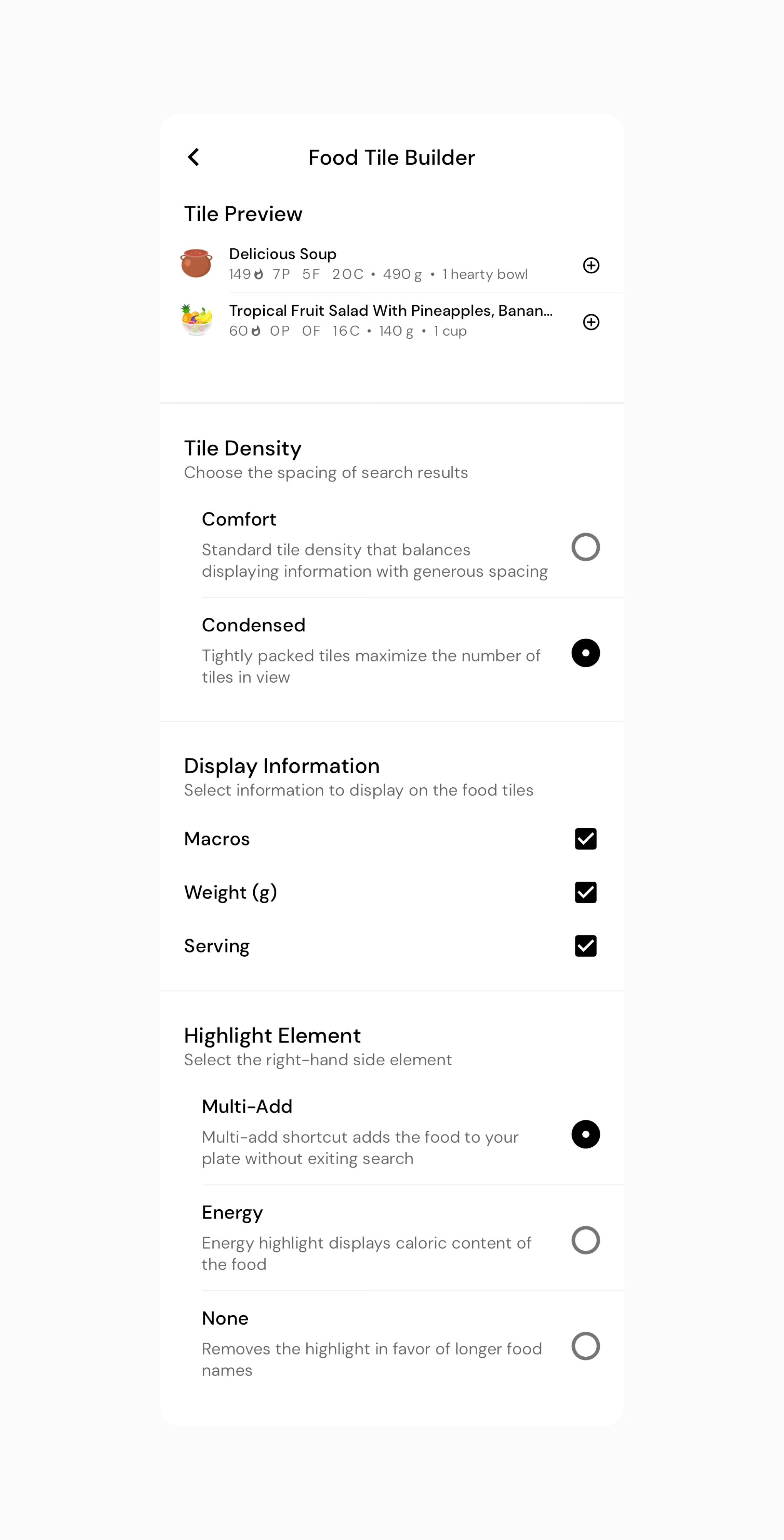Here is a cleaned-up and detailed caption:

---

Screenshot of a nutritional management app interface titled "Food Tile Builder." The preview showcases images of a delicious soup and a tropical fruit salad featuring pineapples and bananas. Below these images, there's a section displaying nutritional information, which appears to include macronutrients like protein and calories, though the text is quite small. 

The app interface is divided into four sections. The second section, titled "Density," allows users to select the spacing of search results with options such as "Comfort" and "Condensed." The "Condensed" option is currently selected and described as lightly packed tiles that maximize the number of tiles in view.

Additionally, the app offers a feature to select what information to display, including macros, weight, and serving sizes. The highlighted feature is the "Multi-Add" shortcut, which enables users to add multiple food items to their plate without exiting the search. Overall, the app appears to be designed for weight management and nutritional tracking.